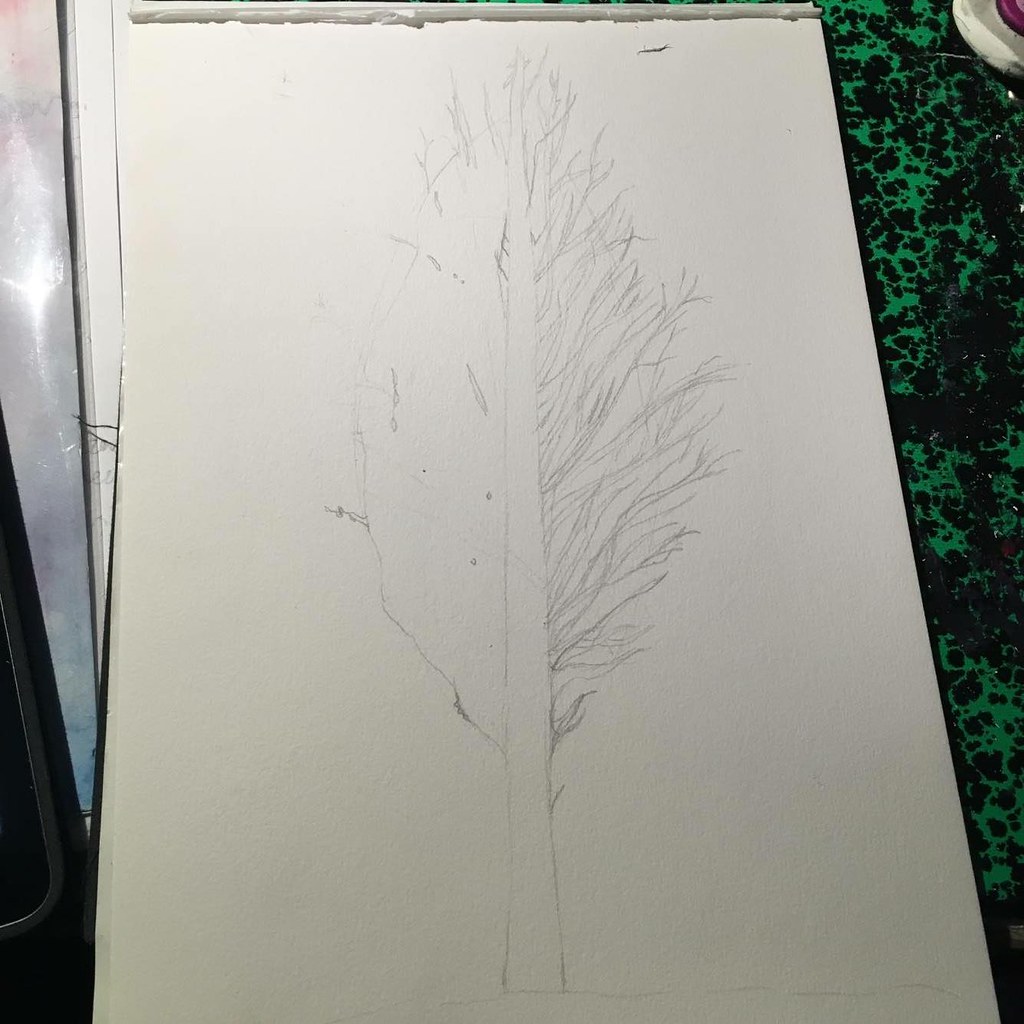This detailed image depicts a mid-process pencil sketch on a piece of thick, high-quality drawing paper, showcasing an emerging tree. The tree spans the entire height of the paper, with its tip touching the top edge and its base near the bottom. The left side of the tree features a lightly sketched outline of leaves in a half-circle, complemented by a few spindly branches, while the right side is more detailed, displaying numerous branches rendered with quick pencil strokes. The trunk is bare and devoid of intricate details like bark, providing a stark contrast to the elaborate branch work on the right. Below the tree, a faint pencil mark suggests the ground from which the tree emerges. 

The paper has been ripped out of a notepad, evidenced by the tear at the top. The scene includes various items in the background: a green and black marbled tablecloth to the right, a black cell phone peeking from the bottom left corner, and some silver-colored reflections on the left side. Additionally, obscure items such as folders or a desk surface are visible behind the drawing paper, and a well-worn sneaker appears in the upper right corner, adding a touch of real-world context to the artistic workspace.